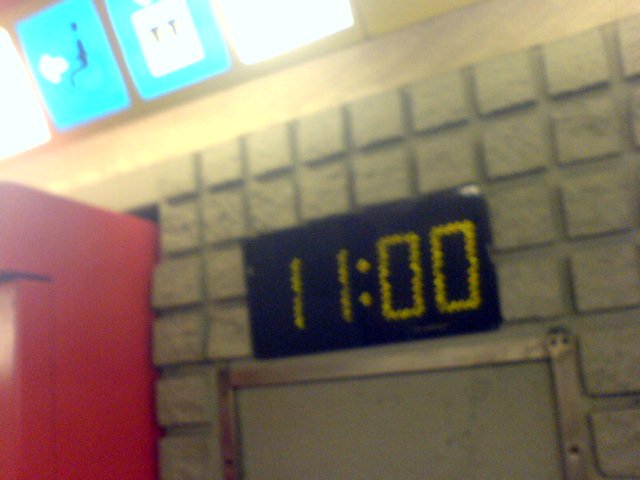The image displays a section of a wall composed of small brick squares arranged in a consistent pattern. Central to the image is a black digital clock showing the time 11:00 in green digits. The clock has a black background and is mounted just above a silver-toned metal frame, which appears to be part of a door frame. To the left of the clock is a shiny red box, though its purpose is unclear. In the background, there are blue and white squares, with one blue square featuring a white inset marked by two vertical lines. The wall itself appears gray due to the lighting, contrasting with the black clock and the vivid colors of the additional elements.